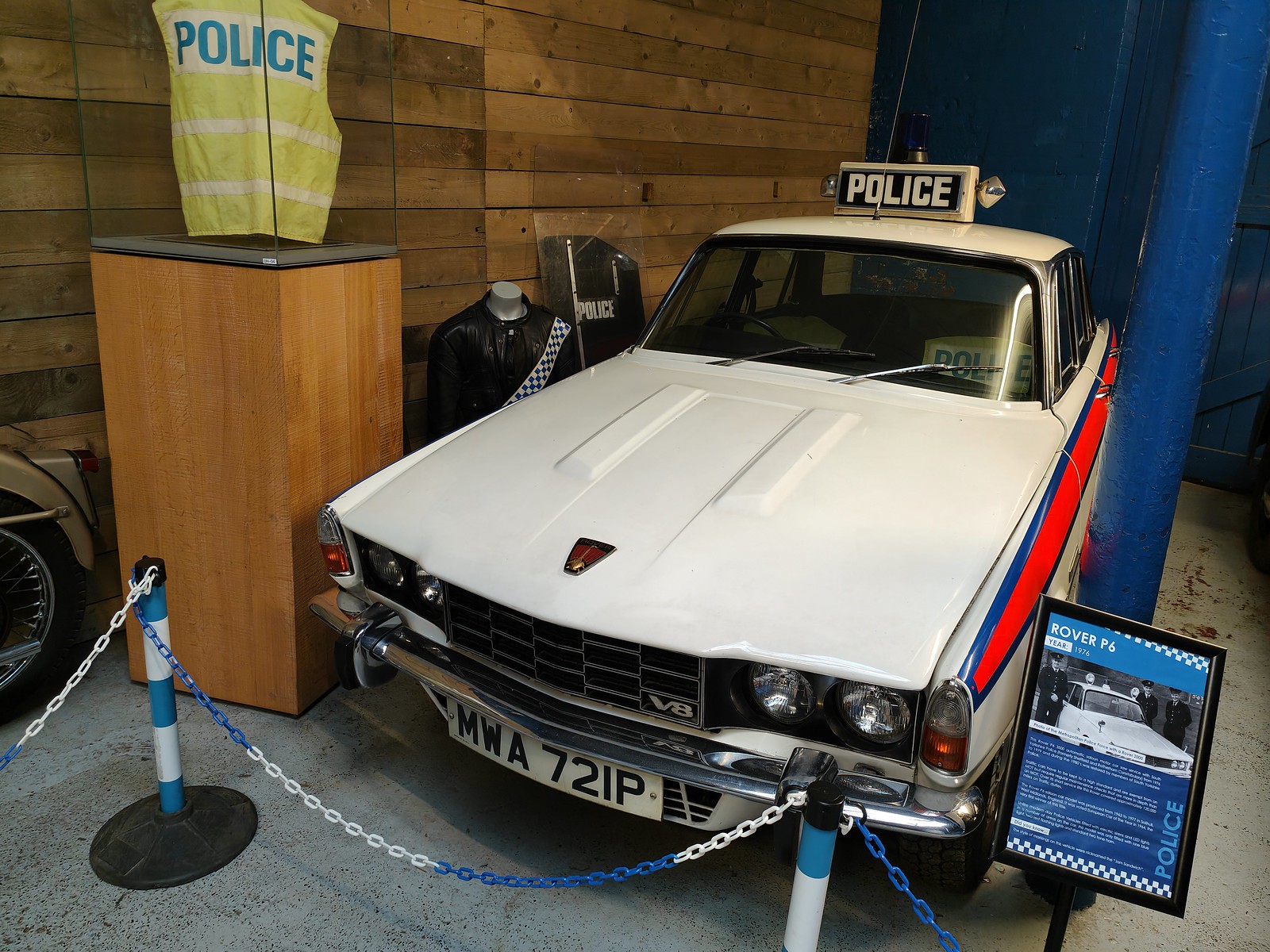This detailed photograph captures an exhibit of an antique police car, specifically a Rover P6, prominently showcased in a museum setting. The vehicle, dating from the early 1970s and featuring a distinctive V8 engine indicated by the badge on its grille, bears the license plate MWA 72IP. The white car, adorned with red and blue stripes along its side panels, also sports a traditional black and white "POLICE" sign mounted atop. Flanking the front of the car, a blue and white chain barrier indicates the display boundaries.

Adjacent to the car, on the right, stands a sign on a metal stand featuring the title "Rover P6" and what seems to be the year "1976" along with historical information, though the smaller text remains unreadable. To the left of the car, various police apparel items are encased in glass. A blue and yellow reflective police jacket with "POLICE" in blue letters is displayed in a glass showcase box. Another police uniform, a black torso mannequin complete with a black and white checkered band and missing a head, is positioned alongside a large black crowd control shield labeled "POLICE" in white.

Behind the car, a wooden wall partially covered by a blue curtain forms the backdrop, creating a dedicated area within the museum for this detailed and historically rich display.